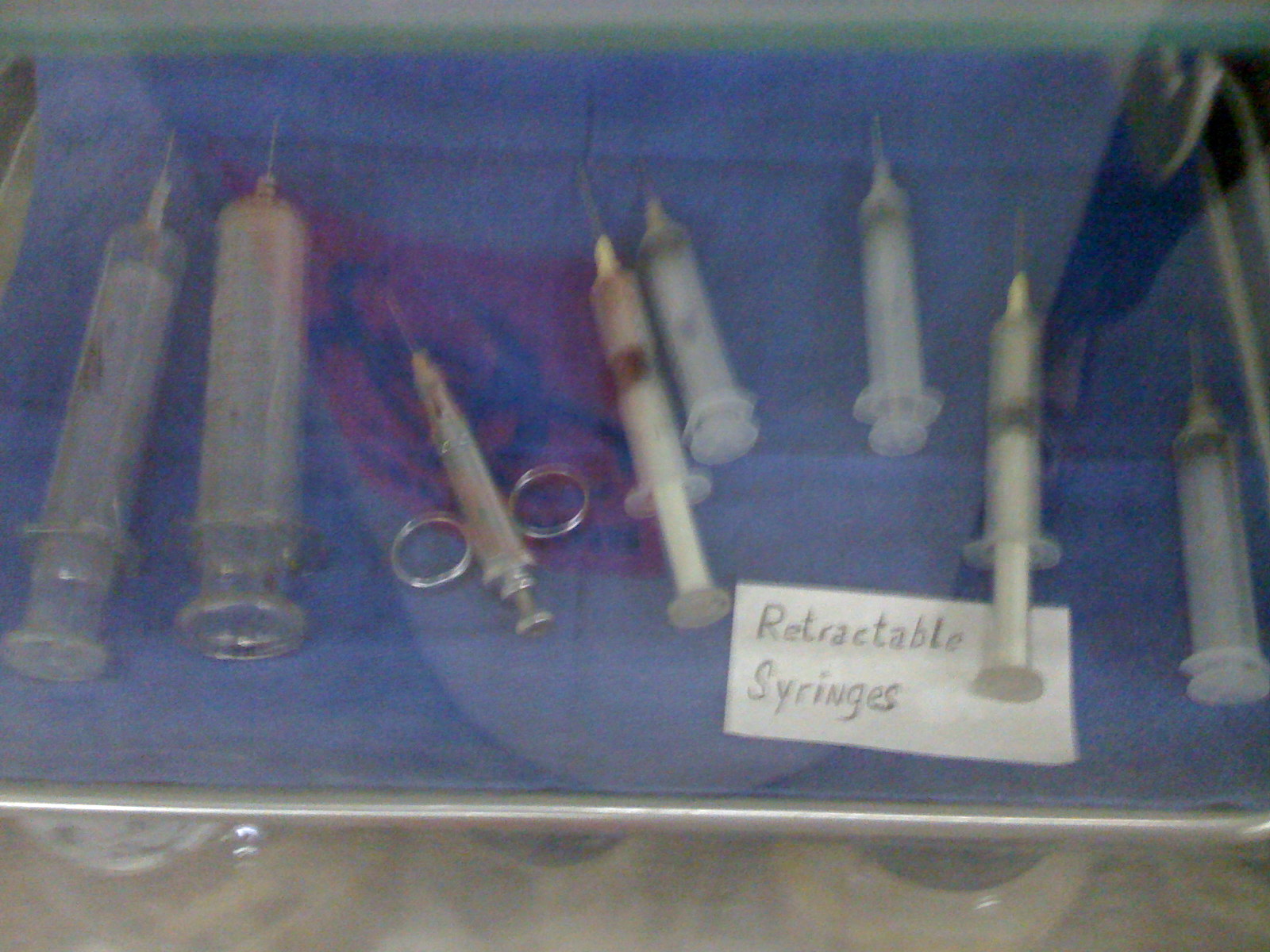The image is a color photograph of very poor quality; it's slightly grainy and soft in focus. Taken from above, it shows a glass display case, evident from the reflections visible on its surface. Inside the display case, there are eight retractable syringes of varying shapes and sizes, suggesting some are older while others are newer. A handwritten note in black pen labels them as "retractable syringes." The syringes are laid out on a blue cloth, inside what seems like a stainless steel medical tray. They are made from different materials including plastic, glass, and stainless steel. One syringe is particularly notable for its design, featuring two metal loops for finger placement to assist in plunging. Reflected in the glass, there is a red background with a black biohazard symbol, hinting at a nearby item displaying this warning sign. The context suggests the syringes are displayed in a medical museum, showcasing the evolution of medical equipment.